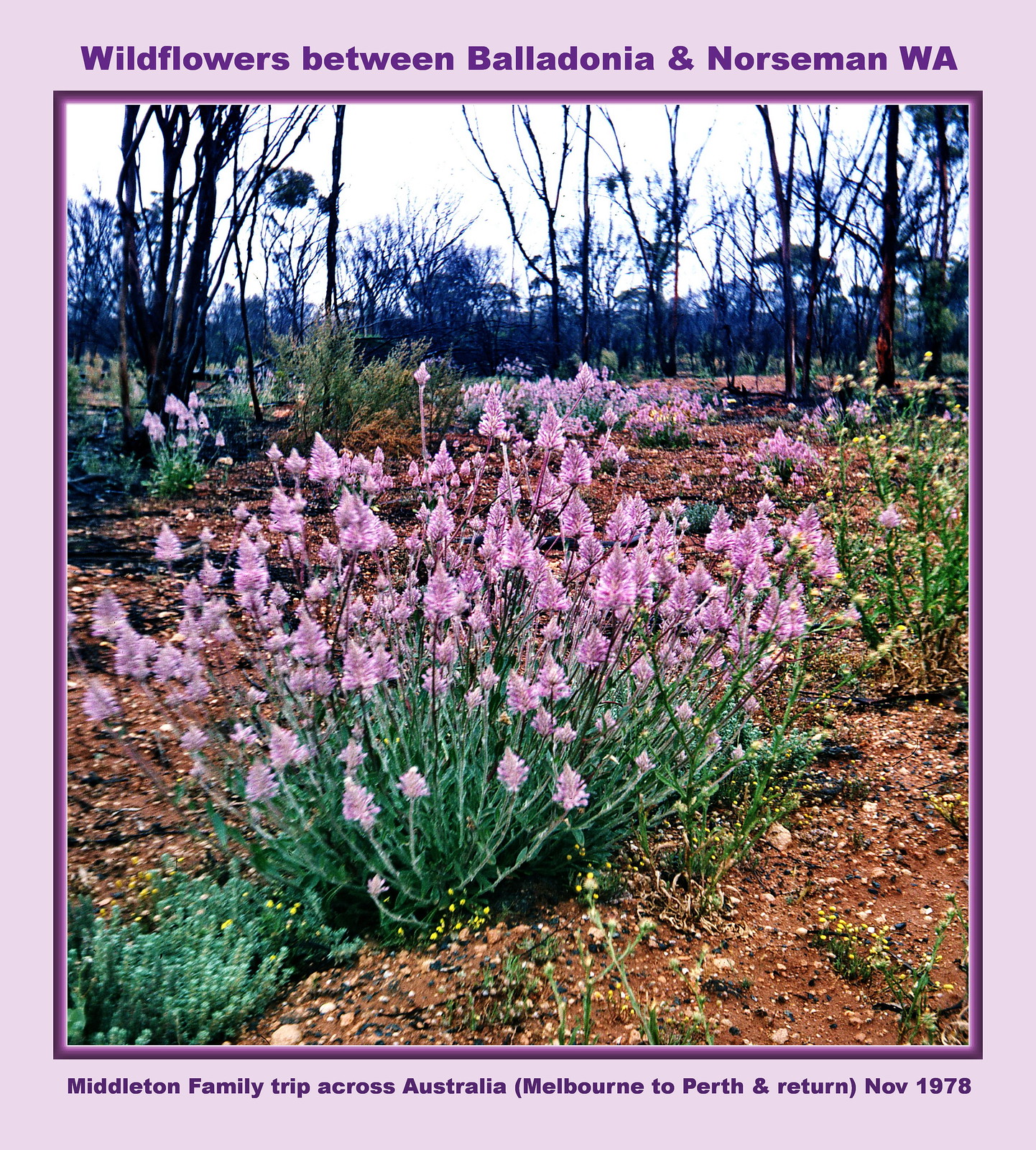The rectangular photograph, measuring approximately six inches tall and five inches wide, is framed by a thin light purple border inset with a darker purple line. At the top, the header reads "Wildflowers Between Baledonia and Norseman, WA" in bold dark purple print, while the footer states "Middleton Family Trip Across Australia (Melbourne to Perth and Return), November 1978," also in bold purple lettering.

Dominating the scene are clusters of green stemmed plants adorned with pinkish-purple flowers, scattered across a rocky, sandy landscape filled with bare, brown spots. As the scene extends backward, a thicket of barren, leafless trees stands against a bright, yet undefined sky that occupies the top third of the photograph. The sense of a winter scene is accentuated by the stark, leafless trees and the cool, grayish-blue hue of the sky, contrasting with the vibrant wildflowers below.